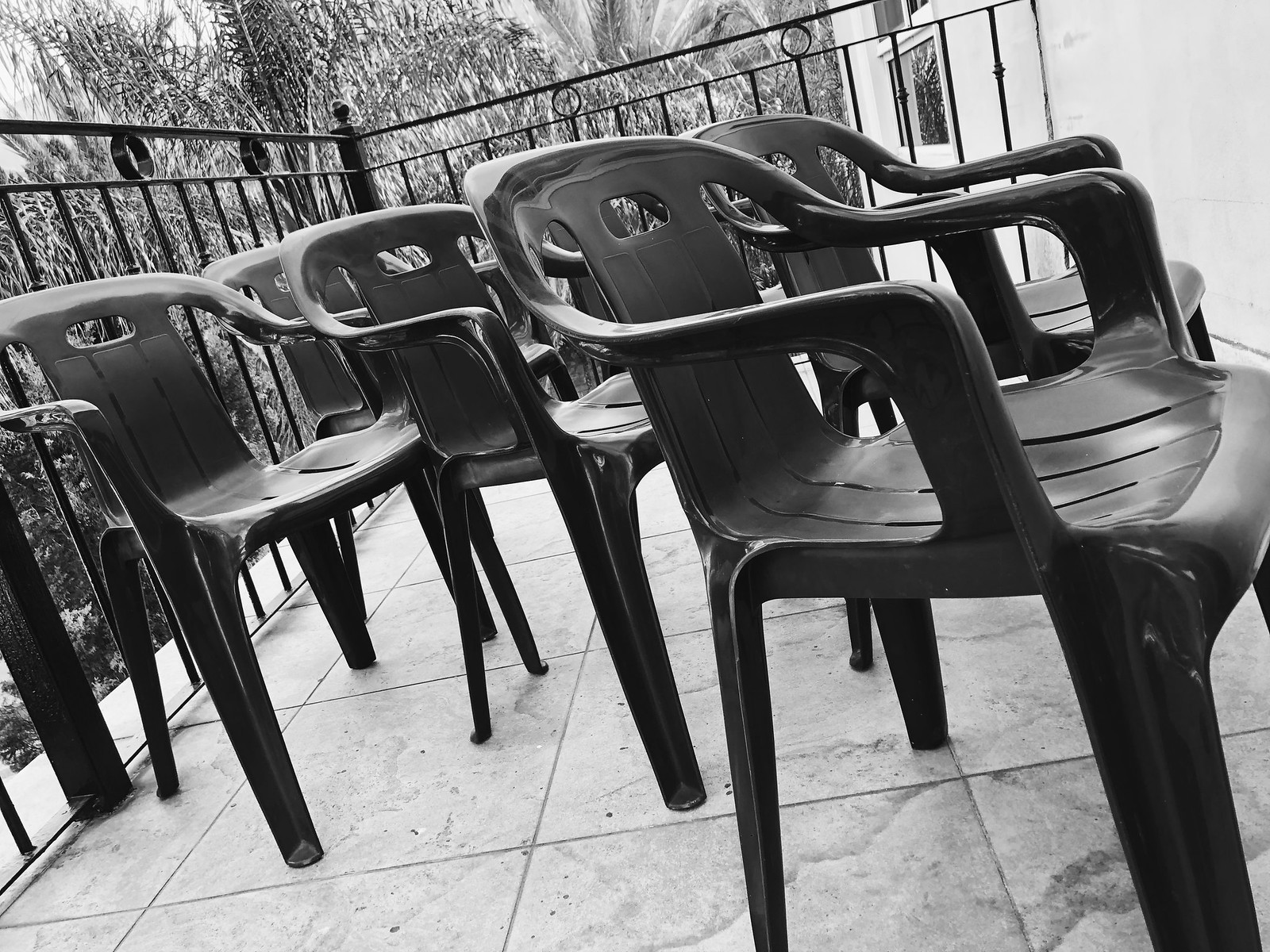This black-and-white photograph captures an outdoor patio or balcony area with a white tile floor and a black wrought iron railing featuring thin vertical uprights and decorative circular patterns. The focal point consists of five dark plastic chairs with curved armrests, open sides, and carrying handles on the backrests. These one-piece, stackable chairs are structured with four legs each and have slits in the seats for airflow and drainage. The chairs are arranged in a somewhat haphazard manner, all facing the right side of the image. On the right, a building wall with a rectangular window can be seen beyond the railing. The background features lush, tropical foliage extending upwards, indicating a natural, verdant setting beyond the confines of the patio.